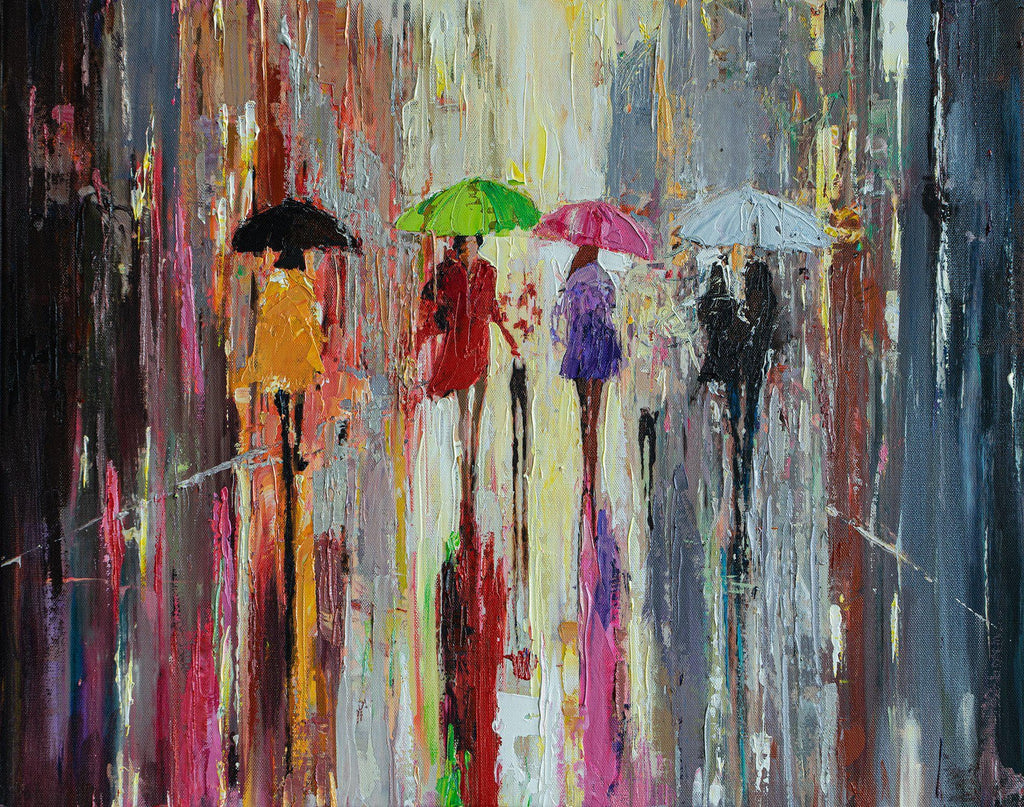The painting depicts a vividly colorful and rainy street scene, rendered in an abstract, impressionistic style with thick, textured vertical strokes likely created using a palette knife. The background features a cascade of descending colors—orange, red, yellow, light and dark blue, and black—contributing to the blurred illusion of rain and a wet atmosphere. At the center, four women with their backs mostly turned are walking along what appears to be an alleyway, each holding a vibrantly colored umbrella: a woman in a yellow poncho with a black umbrella, another in a red jacket with a lime green umbrella, a third with brown hair in a pinkish-purple coat holding a pink and red umbrella, and the last one in black pants and a black jacket with a bluish-gray umbrella, walking toward the viewer. Accompanying them are two small dogs. The lower half of the painting features a smooth, reflective surface, enhancing the sense of pooling water and giving a mirrored effect to the scene above. The artistic use of messy, long vertical lines emphasizes the rainy, abstract nature of the artwork, capturing both motion and tranquility in a bustling, rain-soaked urban setting.